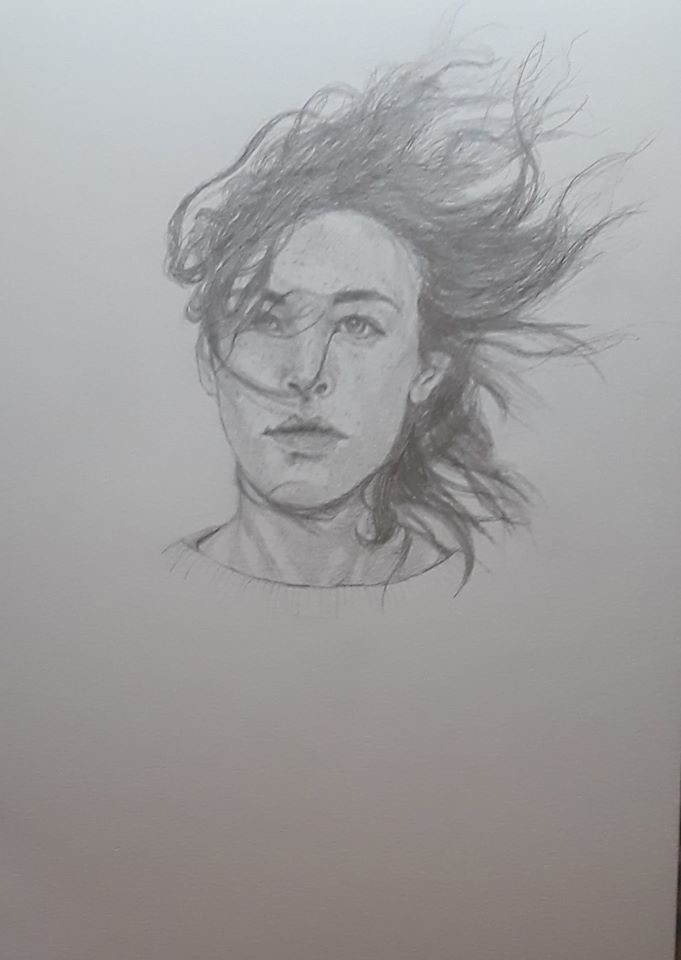This detailed pencil illustration captures the face of a woman with long, dark hair that seems to be blown by the wind, causing a portion of it to obscure part of her face. Despite the monochromatic black and gray palette, the artist masterfully renders the depth and texture of her hair and facial features. Her eyes, also rendered in shades of gray, remain enigmatic in the absence of color, while her expression is notably serious, conveying a sense of introspection or melancholy. The drawing extends just below her neck, revealing the simple collar of a shirt, but goes no further, leaving the focus entirely on her face and hair. Set against a stark white background, the portrait stands out with striking contrast, emphasizing the meticulous detail and shading of the pencil work.